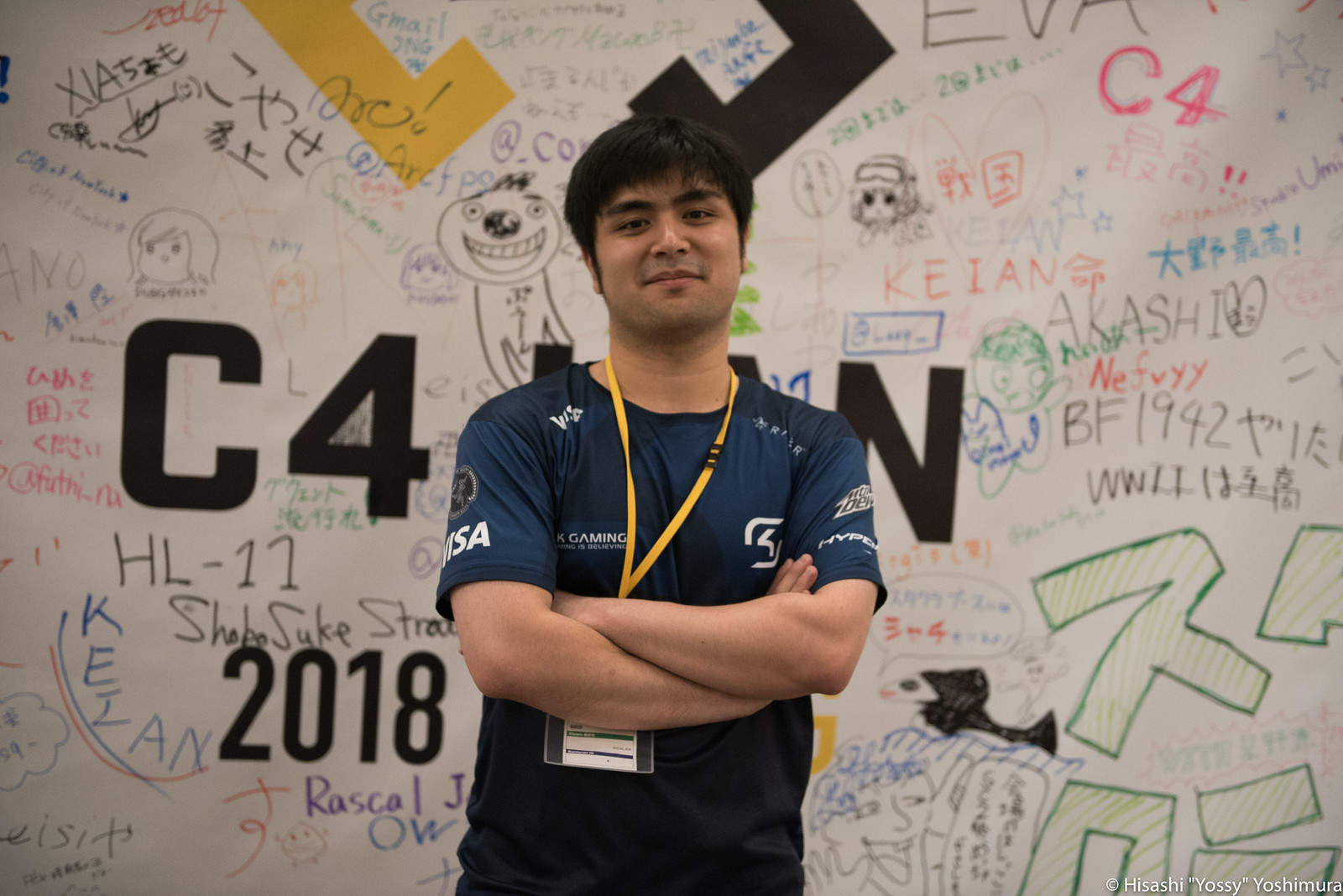In the image, a younger man, potentially in his twenties and of Asian descent, stands against a white background that resembles a poster board filled with colorful markings and doodles. He has straight black hair styled flatly to his eyebrows, thick eyebrows, and a clean-shaven face, giving him a smirking expression. He wears a navy blue athletic jersey, which is suggested to be a gaming jersey, and it features a Visa sponsorship. His arms are folded across his chest, and he has a yellow lanyard around his neck with a name tag in a plastic holder. The background is a whiteboard-like surface with various drawings and scribbles in blue, black, red, green, and yellow hues. Dominating the background are bold black letters, possibly made from tape or digitally printed, that spell "C4" and "2018," hinting at a conference setting.